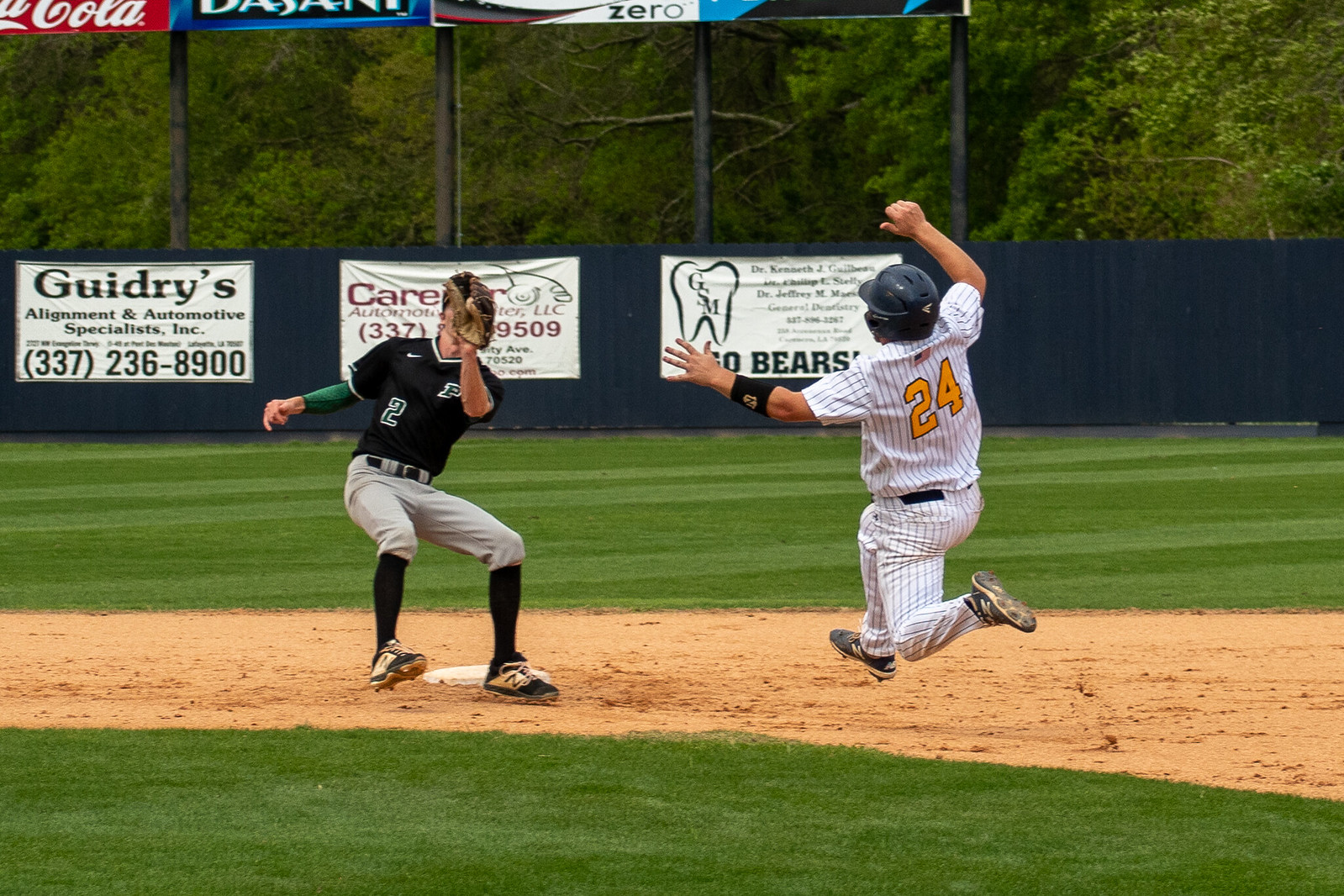This detailed color photograph captures an outdoor daytime baseball game. The central focus is on two players engaged in a play at what seems to be second base. The player in the foreground, wearing a gray and green uniform, gray pants, a black shirt, black socks, and a green arm sleeve, is number 2. He stands right above the base, his mitt covering his face as he either has just caught or is about to catch the ball. The other player, dressed in a white pinstriped uniform with a large yellow number 24 on his back, is mid-air, just about to slide feet-first into the base. He sports a blue batting helmet. Surrounding the field, there are lush green trees, adding a verdant backdrop to the blue-fenced boundary of the baseball field. Three white banners adorn the fence: one for "Guidry's Alignment Automotive Specialists" in green text, another partly visible for "CARE Automotive" in red text, and the third one with a tooth logo reading "G.S.M. Go Bears." Further advertisements for Coca-Cola, Dasani, and something labeled "zero" punctuate the scene, contributing to the lively atmosphere of a sports game.